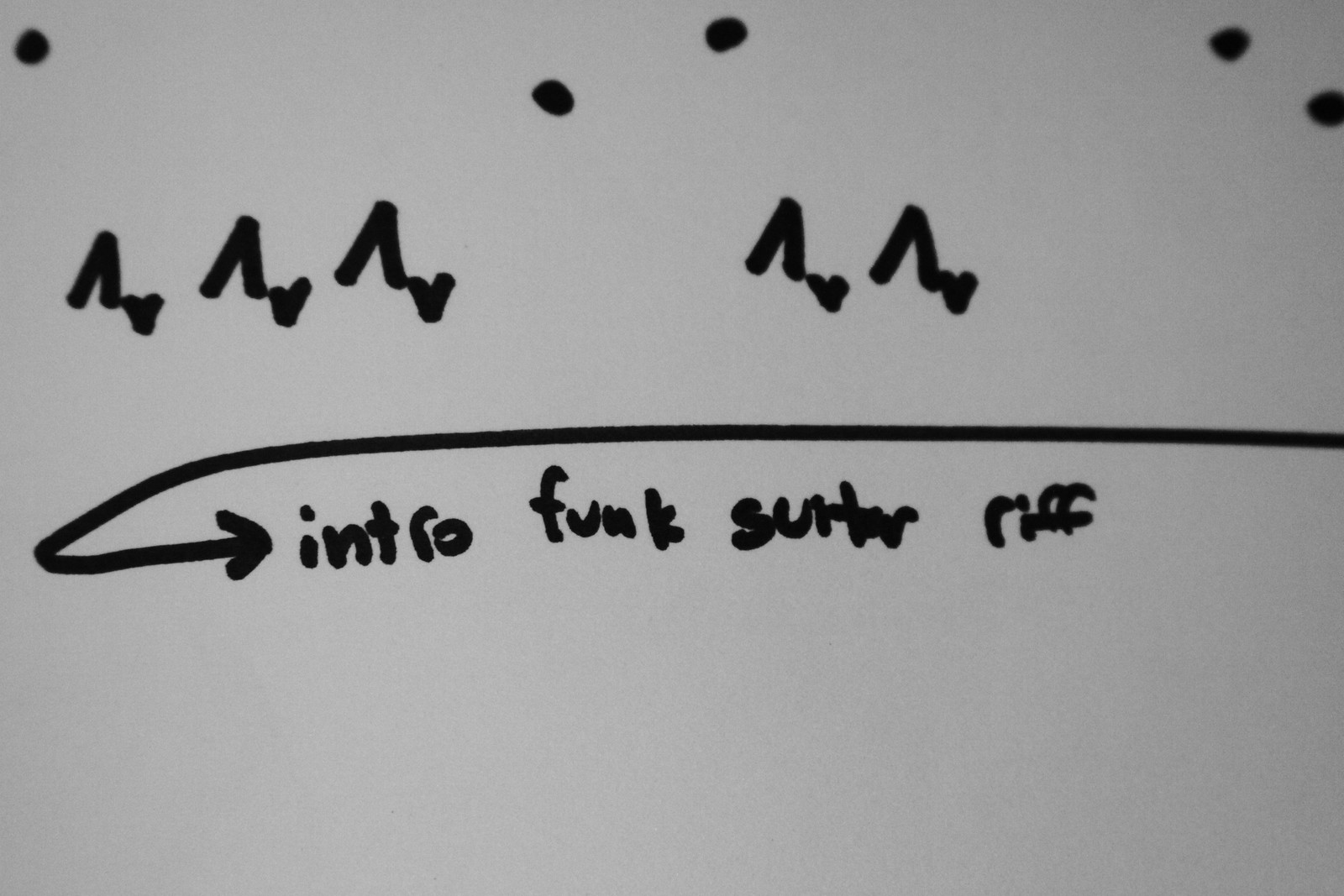This photorealistic image captures a white sheet of paper featuring handwritten text, designs, and symbols in black marker. Dominating the scene is an arrow that starts from the right side of the page, loops across the center towards the left, and then doubles back to point at the beginning of a handwritten sentence just below the center of the page. The sentence reads "intro, funk, surfer, riff." Above the arrow, a series of intricate designs composed of an uppercase A paired with a smaller upside-down A appear. These paired A symbols are arranged in a pattern: three near the left side and two just to the right of the center. Additionally, six black dots are scattered across the page: two in the top right, two in the middle, and one each on the left and right sides. This meticulously constructed layout resembles a graph, chart, or a musical notation, offering a glimpse into a creative or instructional schematic.